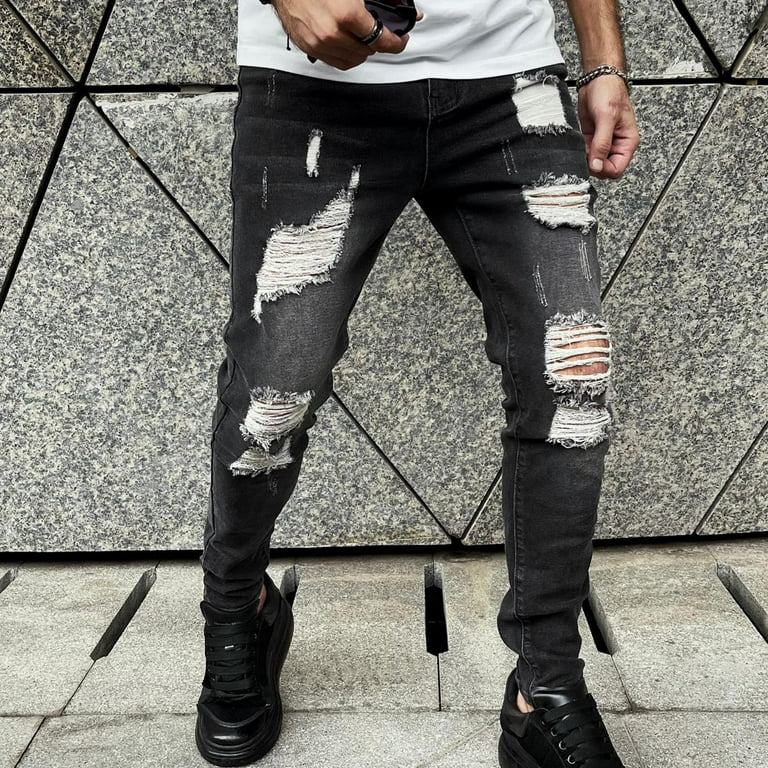This is a vertical rectangular image of a male model’s lower half, standing on a sidewalk composed of concrete blocks that form a grate-like pattern for drainage. Behind him is a textured black and white granite wall, where each piece is cut into a triangular shape to create a distinct background. He is dressed in a pair of black, acid-washed skinny jeans that narrow down to his ankles, with intentional distressed holes revealing white threads across the legs. The distressed areas are prominently featured on both thighs and knees. His footwear consists of black low-top sneakers. Although only the bottom half of his white t-shirt is visible, his posture is dynamic: his right foot bears most of his weight while he is on his left tippy-toe, suggesting a casual yet poised stance. One arm hangs at his side adorned with a bracelet, and his other hand is raised in front of him, holding a black object, likely a phone.